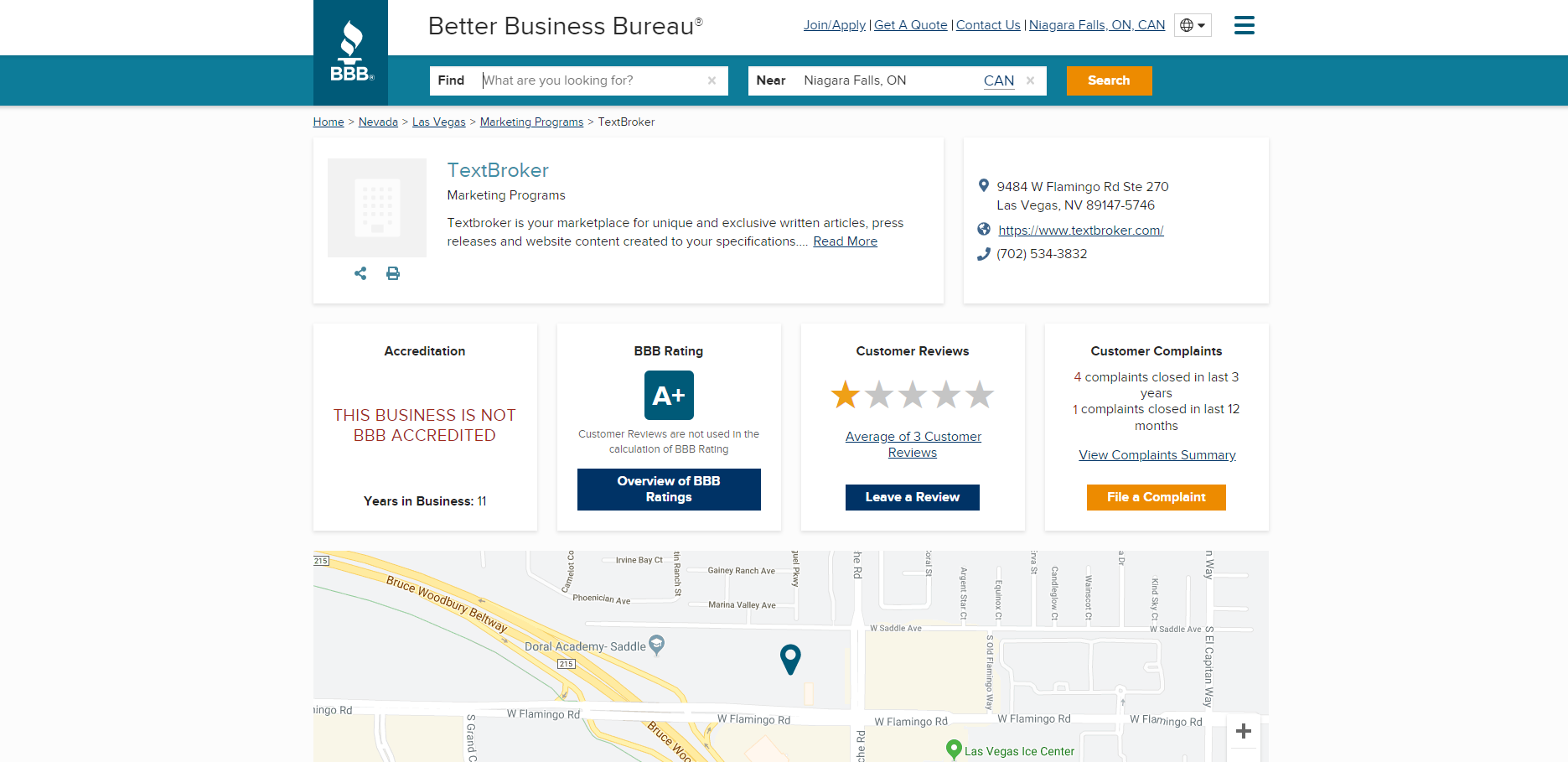This image is a cropped screenshot of a business listing on the Better Business Bureau (BBB) website. 

At the top left corner, there's a blue square housing the iconic BBB logo. To the right of the logo, in small black text, the words "Better Business Bureau" are displayed. Below this section, a blue bar runs horizontally across the top of the page. It features a text box labeled "Find" on the left side, followed by another box labeled "Near," intended for users to input a city, and finally, a "Search" button on the right.

Just below this blue bar, there's an orange bar with a large white box on the left. This box contains a thumbnail image of the business name accompanied by a brief description of the company. To the right of this large white box, there's a smaller white box containing the business’s contact information.

In the middle section of the listing, four horizontally aligned boxes provide specific details about the business. The first box, labeled "Accreditations" in small blue letters, states that "this business is not yet accredited." Next, the "BBB Rating" box displays an A-plus rating inside a blue box. To its right, the "Customer Reviews" box showcases five stars, with only one star lit up, indicating the company’s limited user reviews, and includes a prompt to read the reviews. The final box, labeled "Customer Complaints," includes an orange "File a Complaint" button at the bottom.

The entire lower section of the screenshot is occupied by a map featuring a pin drop to indicate the location of the business.